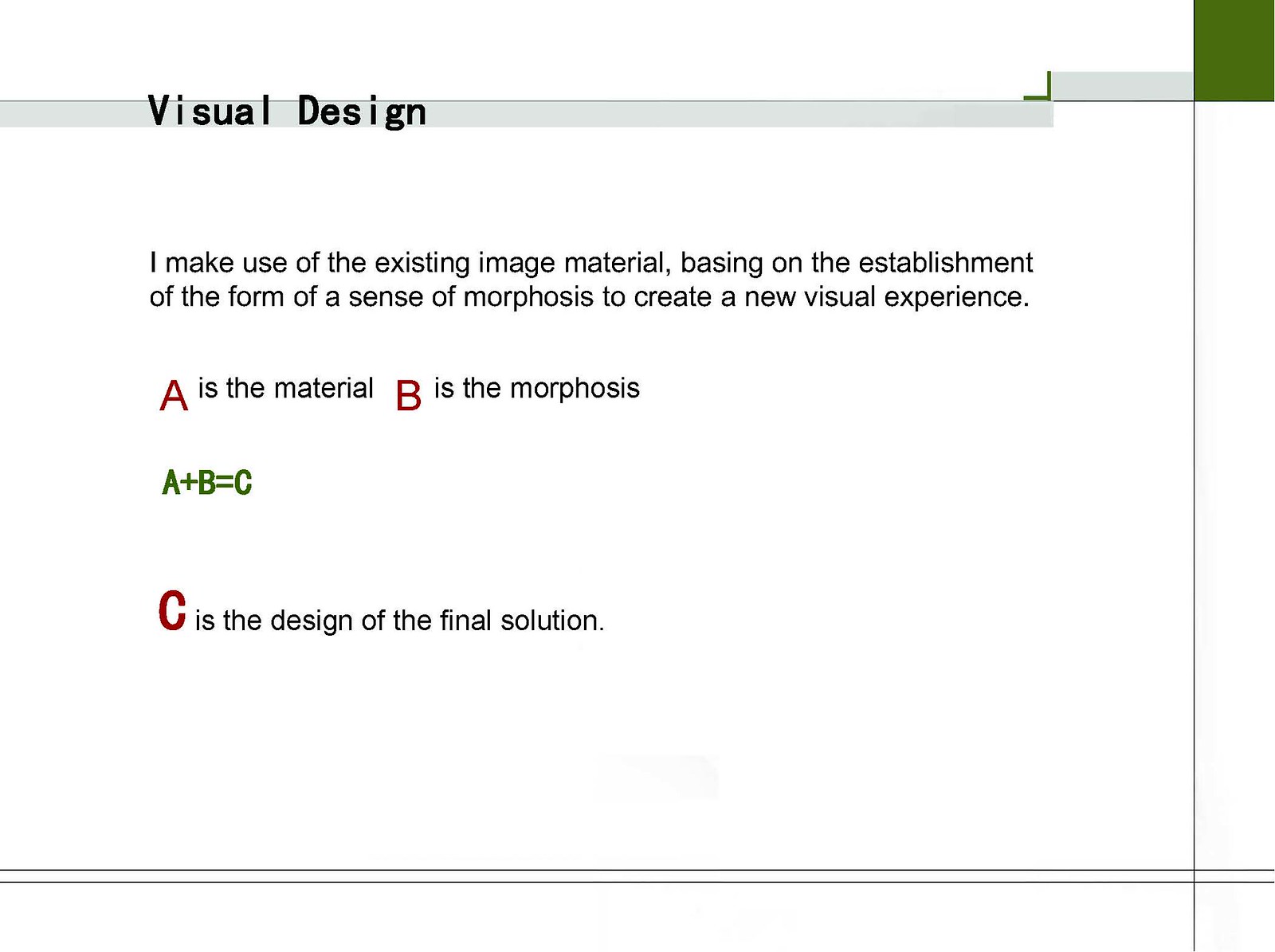The image appears to depict a concept from a visual design course. It features a structured layout on a white background, with a green rectangle positioned in the top right corner. At the top of the image, in bold black letters, it reads, "Visual Design." Directly beneath this header, a passage in smaller text states, "I make use of the existing image material, basing on the establishment of the form of a sense of morphosis to create a new visual experience."

Following the passage, the image outlines an equation central to the concept being presented. In red, capitalized letters, it identifies, "A is the material," and "B is the morphosis." Below these, a green equation reads, "A + B = C," signifying that "C," also capitalized in red letters, "is the design of the final solution."

The color palette includes green, black, grey, white, and red, with a grey horizontal line appearing towards the end of the page. Overall, the image serves as an illustrative rule or principle within the visual design context, demonstrating how material and morphosis combine to form a final design solution.